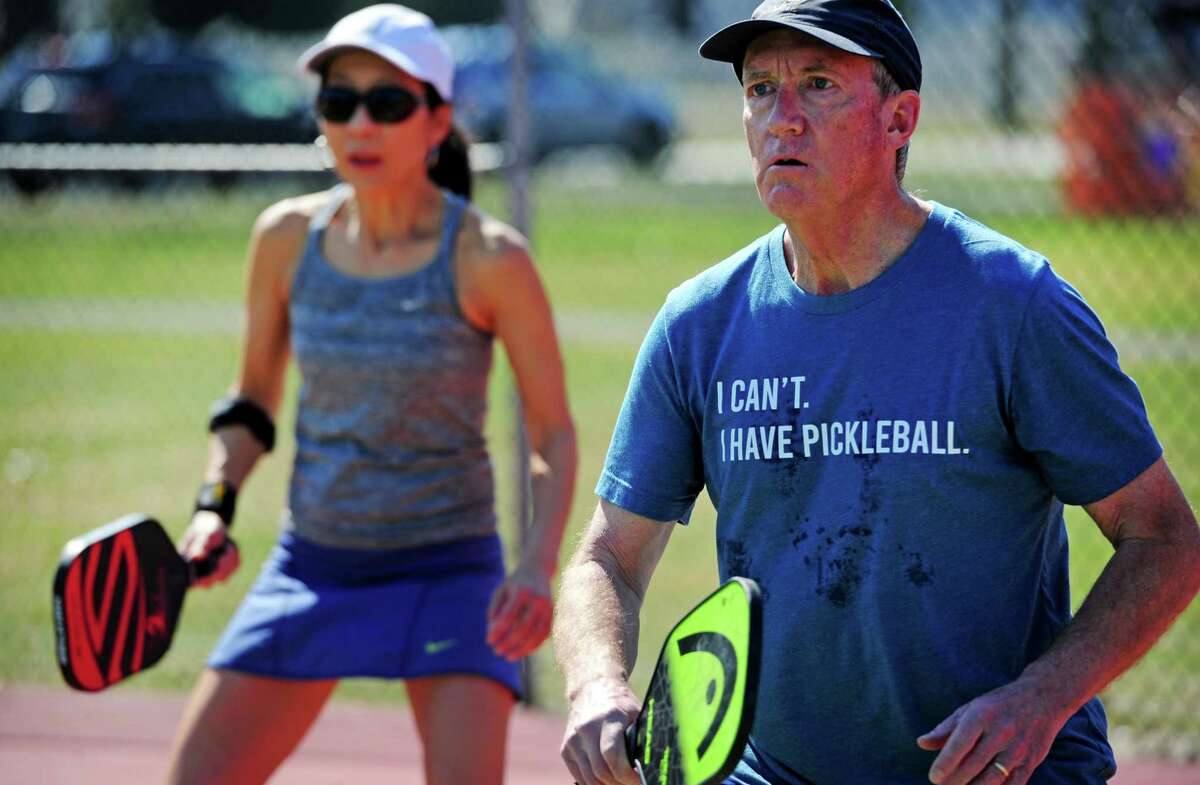The image depicts an elderly couple engaged in a game of pickleball on an outdoor sports court. The man, likely in his 60s, stands on the right side of the image, wearing a black baseball hat and a blue t-shirt that reads "I can't, I have pickleball" in white text. His pickleball paddle is fluorescent green with a distinctive black rainbow shape and a circle beneath it. Opposite him, the woman sports a white baseball cap, dark black sunglasses, a Nike grey tank top, and a blue tennis skirt. She holds a black and orange pickleball paddle in her right hand and is equipped with a wristband and a sweatband for support. Behind them, the court is filled with friends and other players, making for a lively and active scene. The setting is clearly outdoors on a marked sports court, captured in a horizontal rectangular photograph. The colors in the image are diverse, featuring shades of blue, neon green, grey, black, and white, adding vibrancy to the scene.